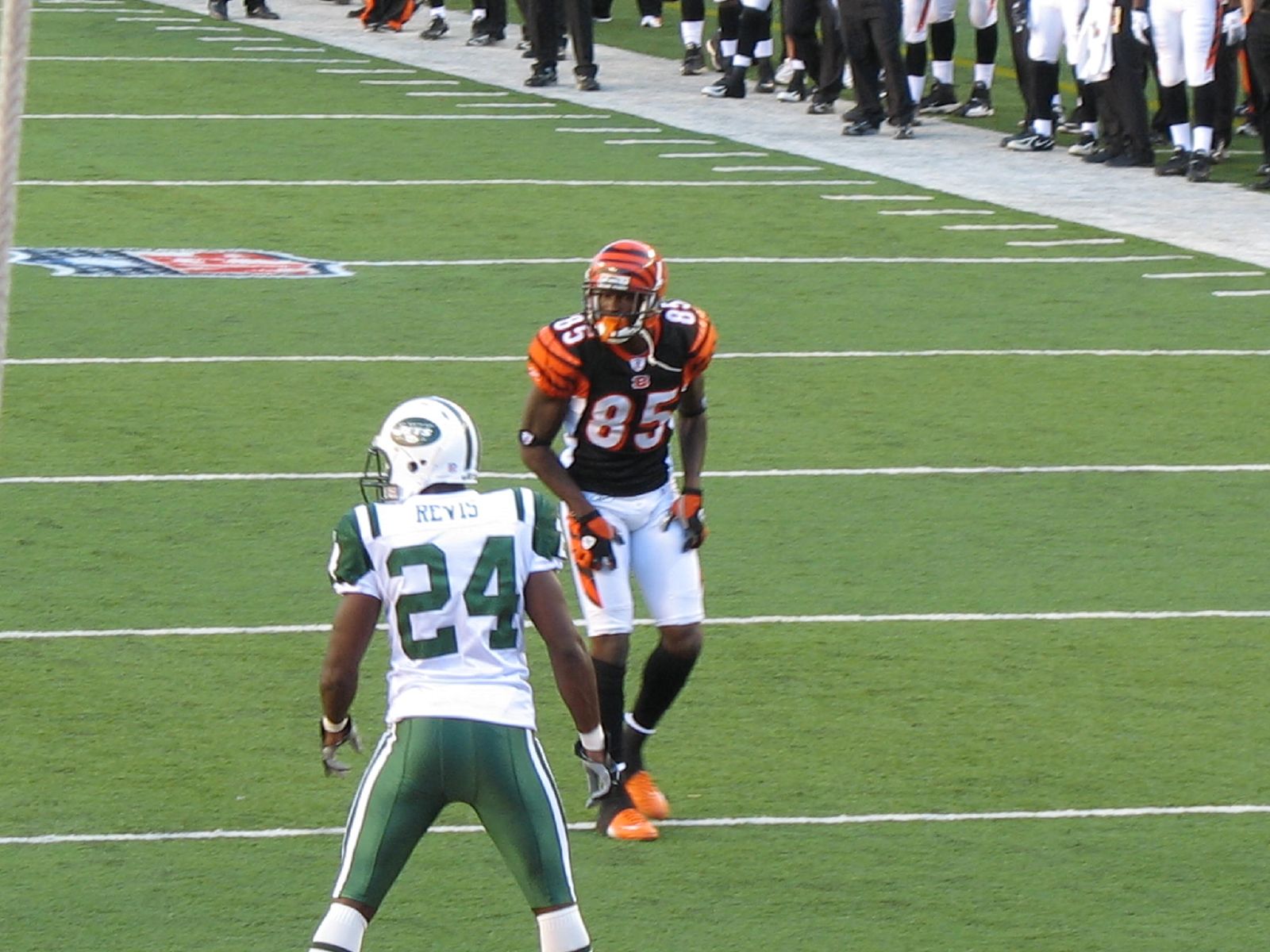The photo depicts a well-maintained green football field prominently divided by white lines, with the iconic NFL shield logo in white, blue, and red visible just above the halfway point on the left side. At the center of the image stand two American football players from different teams. The player with his back to the camera wears green pants and a white jersey with green numbers, displaying "Reyes" and the number 24. In front of him, facing the camera, is a player in a black jersey with the number 85 on his chest and shoulders, orange arm pads, an orange helmet, white pants, and orange shoes. To the right and in the background, a large crowd watches intently, though only parts of their lower bodies are visible due to the image's framing. The scene is brightly lit, indicating it is taken in broad daylight.